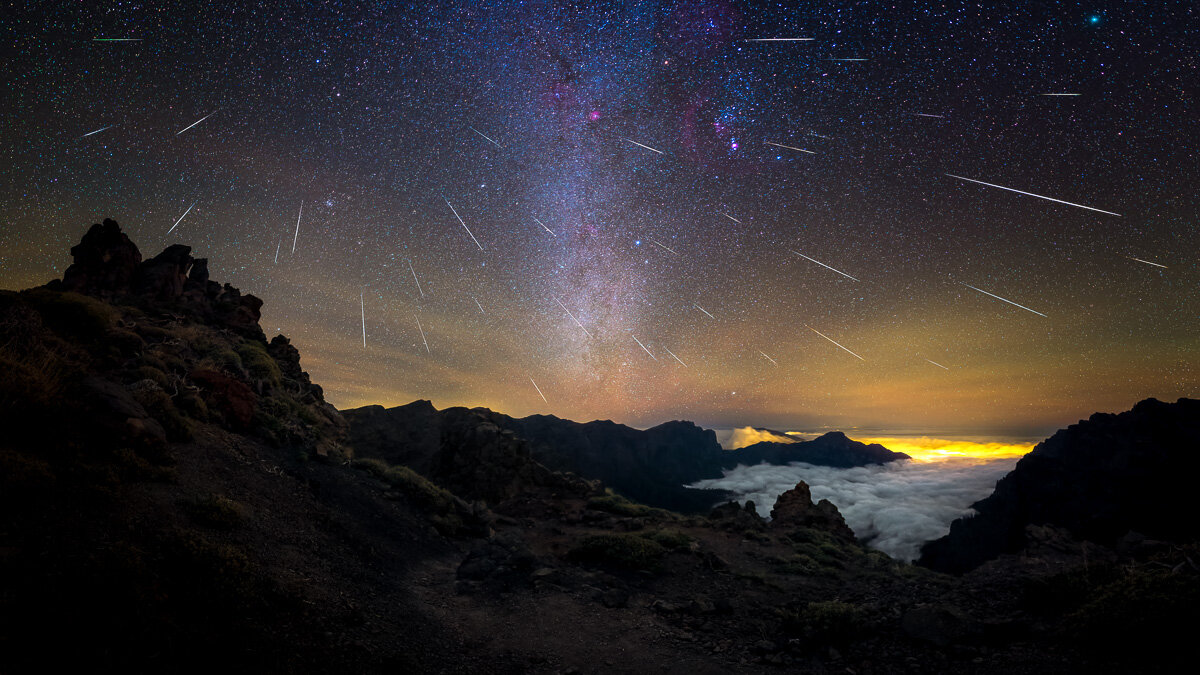This time-lapse photograph captures a mesmerizing nighttime scene set out in a rugged mountain range. The bottom third of the frame reveals nearly black silhouetted rocky peaks with subtle brown highlights where ambient light touches. The mountains are jagged and sharply defined on the top left, gradually smoothing down towards the right. In the distance, another line of darker mountains is faintly visible, separated by a pool of wispy white-gray clouds. These clouds catch a warm, bright orange glow from the distant horizon, indicating the light of a setting sun. Above these clouds, the night sky unfolds in a dramatic display. A slightly brownish lit-up streak of clouds hovers just above the horizon, giving way to a star-studded expanse. The sky is adorned with bright white, pink, and blue dots of stars, and it's dramatically punctuated by numerous white streaks that fan out from the center top left, reminiscent of meteors or shooting stars captured over time. This celestial display, featuring upwards of 15 to 20 streaking lights, creates an ethereal canopy over the serene, mountainous landscape.